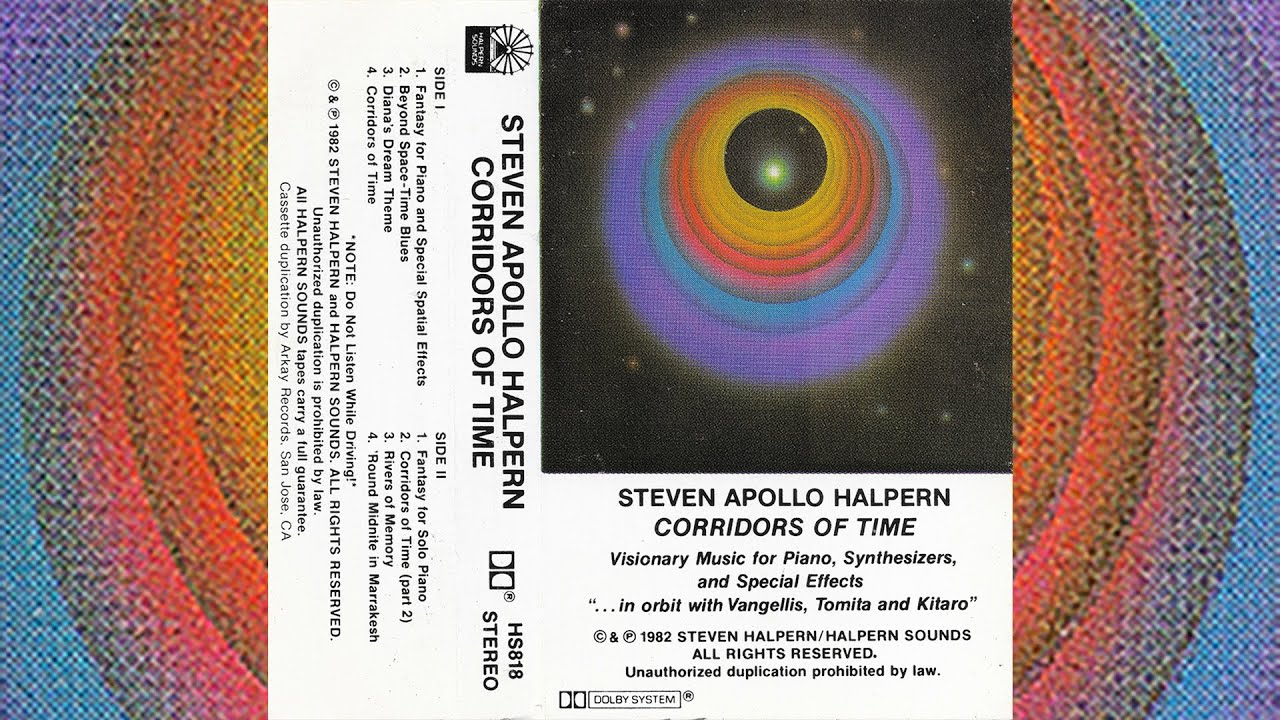The album cover for "Steven Apollo Halperin's Corridors of Time" features visionary music for pianos, synthesizers, and special effects, in orbit with Vangelis, Tomita, and Kitaro. The text is in black and mentions Dolby System stereo sound. The cover art is a stunning abstract of concentric circles in vibrant colors—yellow, red, purple, orange, blue, indigo, and violet—set against a starry background. The stars, scattered throughout the sky, come in shades of red, light green, and blue, creating an ethereal cosmic scene. The bottom of the cover notes "1982, Steven Halperin Sounds, all rights reserved, unauthorized duplication prohibited by law."